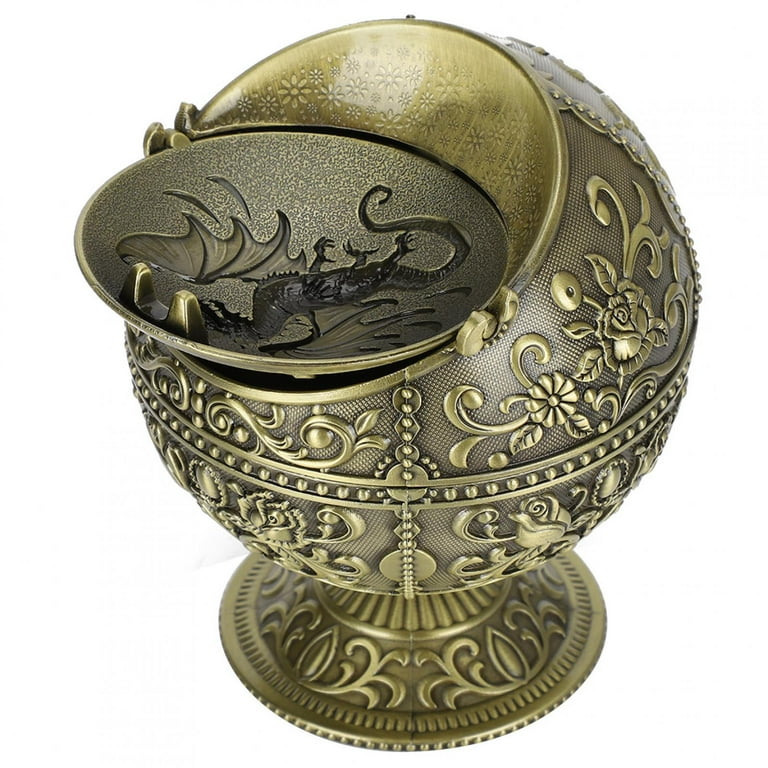This detailed photograph showcases an ornate, globe-shaped ashtray, featuring intricate floral designs with motifs of roses, daisies, and swirling leaves, all brass or bronze in appearance with gold accents. The external surface, resembling a fine basket weave texture, is decorated with curled stems, leaves, and dotted patterns that span the entire sphere. The ashtray is set on a golden plate-like stand and there is an indentation at the top where a section of the globe, adorned with an engraved dragon, flips open to reveal a resting spot, likely for a cigarette. This top piece can be flipped back over, completing the spherical design. The interior of the indentation also contains smaller floral decorations, enhancing the lavish aesthetic of the piece.